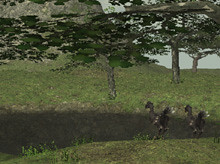The image appears to be a computer-generated graphic, possibly from a video game or created by a graphics program. It showcases a natural landscape featuring a grassy foreground with some weeds, leading up to a shadowy or darker strip that may represent a valley or a creek dividing two sections of land. In the lower right corner, two dark-colored birds, possibly turkeys or vultures with shades of black, brown, and white, are visible. Scattered around are several trees with distinct brown trunks and leafy canopies that suggest an older, less detailed generation of graphics, allowing visibility through the foliage. The background is dominated by a large mountainous or rocky hill that extends above the top left corner of the image, adding depth and a sense of rugged terrain to the scene.